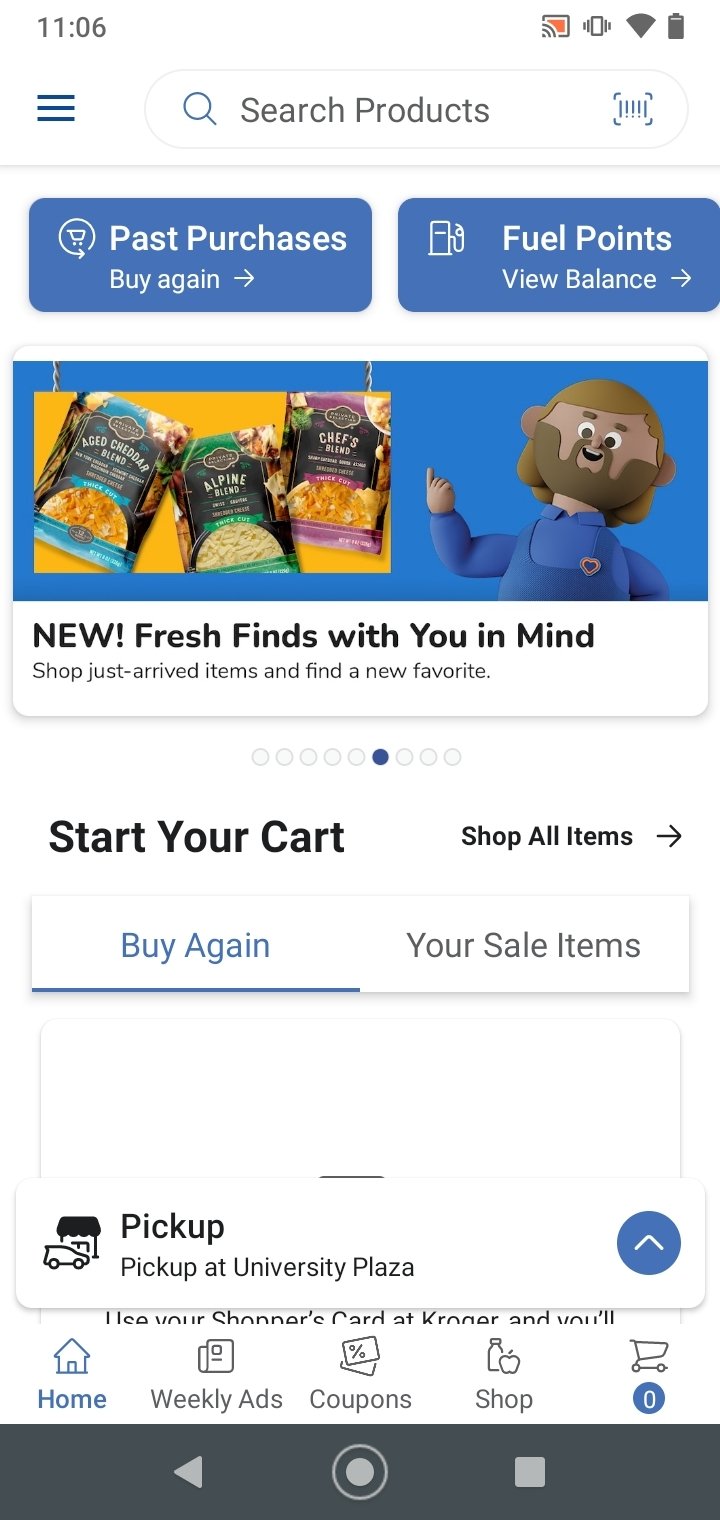The image features a detailed view of a smartphone screen displaying a shopping application interface. At the top of the screen, the time is shown as 11:06, alongside several indicators including Wi-Fi signal strength and battery percentage.

Beneath this, there is a prominent search box with a blue magnifying glass icon labeled "Search Products." Adjacent to the search box is an icon resembling a barcode scanner, suggesting it can be used to check specific items.

The interface also includes several action buttons. One of them is labeled "Past Purchases" with a "Buy Again" option on a blue background. Another button reads "Fuel Points" with a "View Balance" label, accompanied by a fuel tank icon.

A section titled "New Fresh Finds with You in Mind" highlights recently arrived items, encouraging users to discover new favorites. This section showcases various products such as the aged cheddar blend, outline blend, and chef's blend. It features a character with a beard, who resembles a puppet and is pointing to something on the screen, all set against a blue background.

Further down, there is a "Start Your Cart" section where users can shop all items, as well as a "Buy Again" section for previous purchases. At the bottom of the screen, a logo indicates "Pick Up at University Plaza."

The bottom navigation bar includes various tabs such as "Home," "Weekly Ads," "Coupons," "Shop," and an icon representing an empty cart.